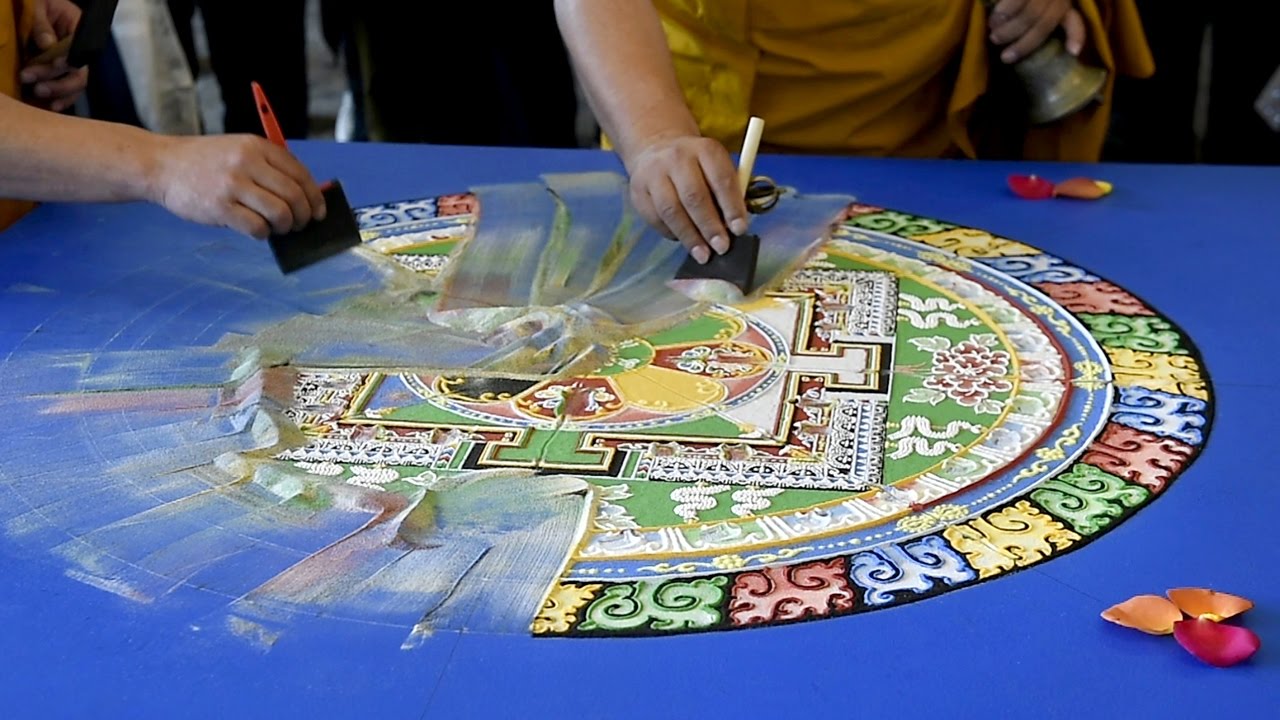The image showcases a horizontally oriented blue table adorned with an intricate and colorful mandala-like design, created possibly with powders. The design features vibrant hues of red, blue, yellow, and green, and includes patterns reminiscent of the New Orleans Saints logo and serpent motifs, surrounded by cloud-like illustrations. The artwork is positioned in a circular layout and appears to be beautifully decorative. Scattered around are shell-like shapes and flower petals, contributing to the ornamental aesthetics. In the scene, two individuals, one wearing a yellow shirt, are in the act of erasing parts of this elaborate design using black eraser-like objects or foam paint brushes. The detailed and dynamic scene suggests a blend of creativity and perhaps transience, as the meticulously crafted artwork is being intentionally brushed away.